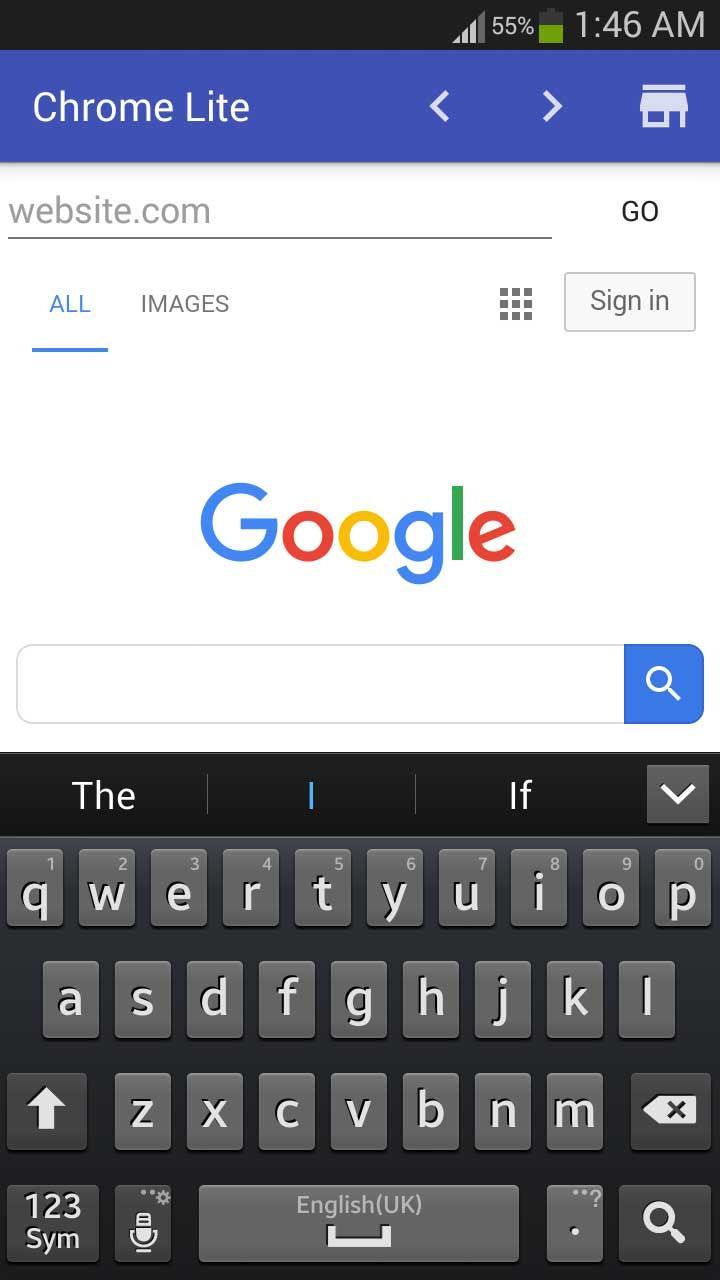The image is a vertically-oriented rectangle with a long side running from top to bottom. At the very top, there is a black border displaying key status indicators. On the right side of this border, you can see a cell phone signal strength icon showing three to four bars, the battery is at 55%, and the battery icon appears to be half-full. The current time, displayed in the same area, reads 1:46 AM.

Just below the black border, a blue banner appears, and in the center of this banner, in white text, it reads "Chrome light." Moving down to the middle section, there is an arrow pointing to the left followed by some more arrows pointing to the right, alongside an unrecognizable symbol.

The middle section switches to a white background displaying "website.com" followed by a thin black line beneath it. On the far right of this line is a button labeled "Go." 

Dropping further down, the interface shows two tabs: "All" in blue with an underline and "Images" written next to it in black text. Adjacent to these tabs on the right side, there is a grid icon resembling a 3x3 matrix, similar to a Rubik's cube. Further to the right is a gray box with a darker gray border containing the words "Sign in."

Below these tabs, the word "Google" is prominently displayed, followed by an open white search box. On the right side of this search box, there is a blue button with a search icon inside, intended for initiating a search. The image concludes with a keyboard visible at the bottom of the screen.